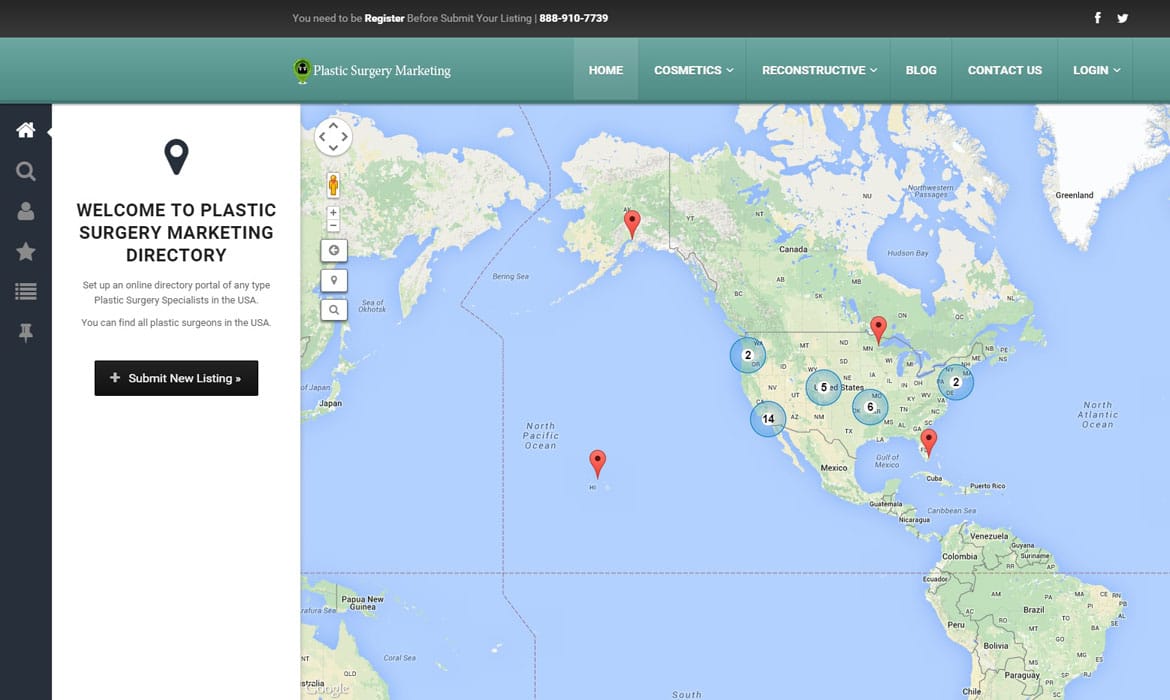The image in question appears to be a web page related to plastic surgery marketing in the United States. At the top of the page, there is a prominent black box with the text: "You need to be registered before submitting your listing." Below this is a green box labeled "Plastic Surgery Marketing." The navigation bar includes options such as Home, Cosmetics, Reconstructive, Blog, Contact Us, and Log In.

On the left side of the page, a section titled "Welcome to Plastic Surgery Marketing Directory" invites users to set up an online directory portal specifically for plastic surgery specialists in the United States. It emphasizes that users can find all plastic surgeons across the country. Below this is another black box with the text: "Submit New Listing."

The page also features a map of North America, including parts of Canada, the United States, and a portion of Africa. This map highlights various locations where plastic surgeons are located. Notably, there are markers in states like Florida and Minnesota, with one erroneously placed in the ocean, suggesting a potential error unless a cruise ship offering plastic surgery services exists, which is unlikely. This map aims to give viewers a visual representation of the distribution of plastic surgery clinics and specialists. Overall, the map is well-detailed and provides valuable information.